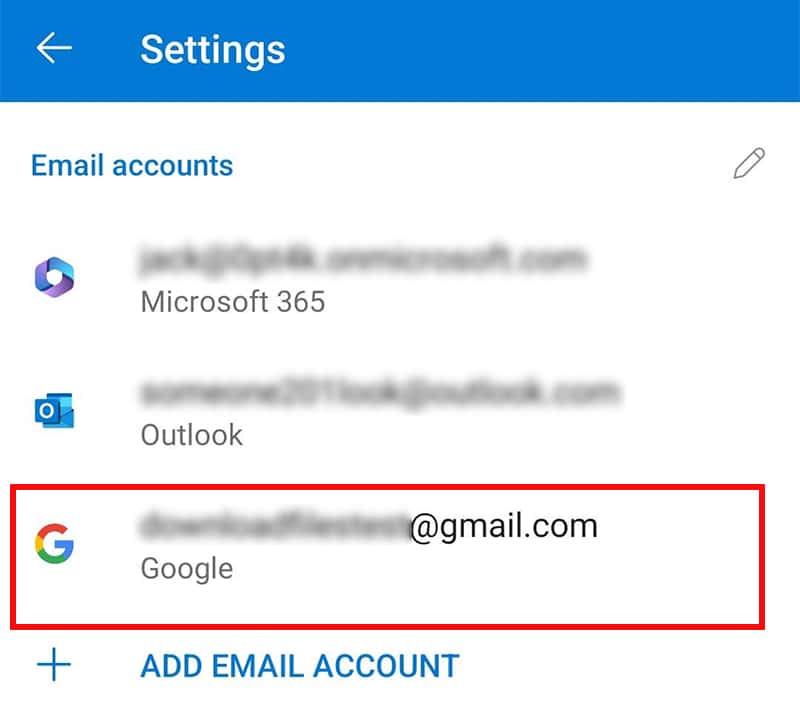This is a screenshot of an email account settings page from a web application. At the top, there is a blue bar with the word "Settings" written in white text, accompanied by a white arrow pointing to the left. 

Below this, "Email Account" is prominently displayed in blue font. To the right of this text is a pencil icon, indicating the option to edit settings. Under the email account section, there is a reference to "Microsoft 365," written in gray font, alongside the Microsoft logo, which features a blue and purple circular pattern.

Further down, the recognizable Outlook symbol for Microsoft Outlook appears, with "Outlook" written in gray font. Nearby, the Outlook folder is depicted with the letter "O." Additionally, the Google symbol, characterized by a red, yellow, green, and blue "G," is present, with "Google" highlighted by a red bar around it. The Gmail email account associated with Google has been hidden or blurred out for privacy.

At the bottom of the screenshot, a plus sign in blue color precedes the option to "Add Email Account," which is written in large blue font.